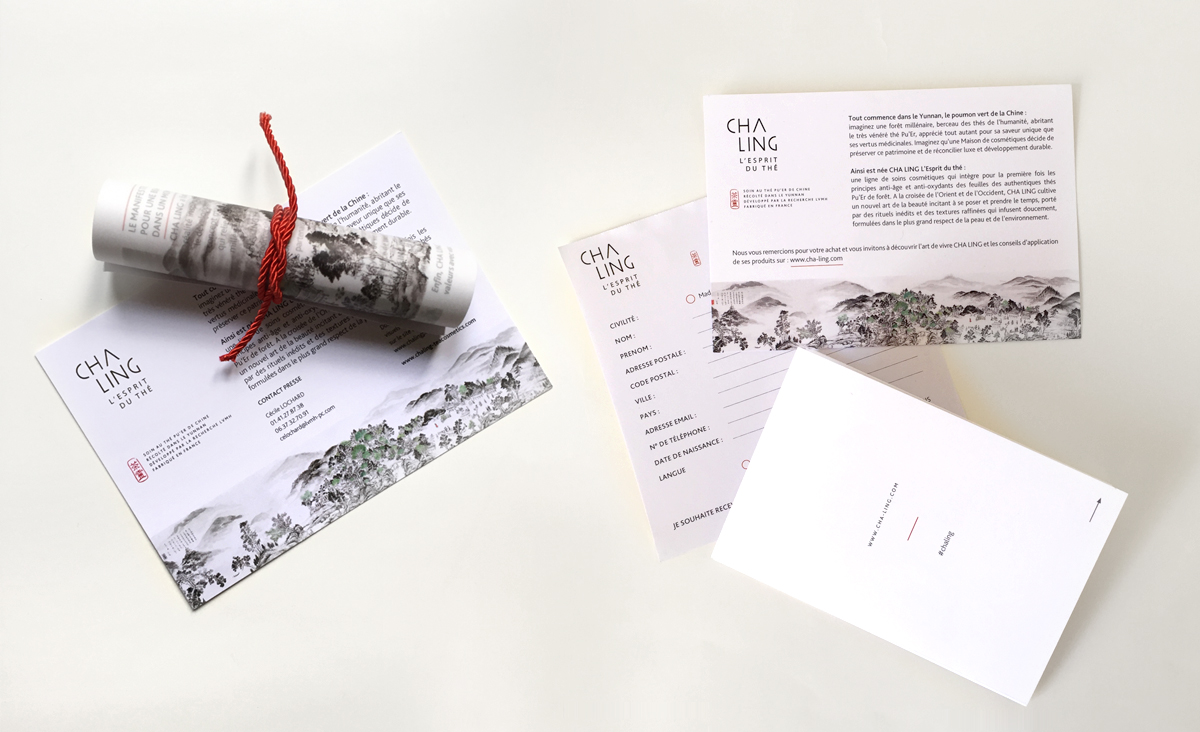The image showcases a display of five artistic cards arranged on a white table, each adorned with the text "Cha Ling" and featuring detailed black-and-white sketches of a mountainous landscape. The cards are positioned at varying angles, including upright, slanted, and upside-down. One notable item among them is a scroll wrapped in intricate, bright red twine, which stands out distinctly against the otherwise monochrome theme. The display likely serves as a storefront or product showcase, with the red twine and occasional red icons on the cards drawing significant visual attention amidst the elegant, traditional imagery. Although the small text on the cards is in another language and not fully legible, elements like postal codes, addresses, or emails are faintly discernible, suggesting a formal or ceremonial context, possibly akin to a wedding invitation.